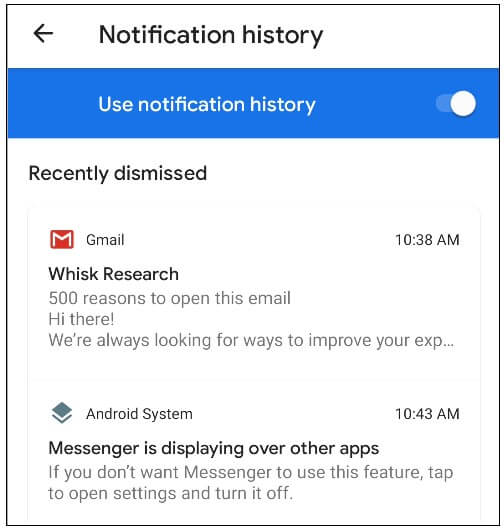Here is a refined and detailed caption for the image described:

---

Screenshot of a mobile device's "Notification History" screen. At the top of the screen, there is a back arrow located to the left, indicating navigation options. Below the navigation bar, a prominent blue rectangular bar spans across the screen with the text "Use Notification History" displayed in white or blue letters, accompanied by a toggle button on the far right.

Directly beneath this bar, the text "Recently Dismissed" is displayed, introducing a section that lists recently dismissed notifications. This section includes two distinct notifications, each contained within white rectangles separated slightly from one another against a white background.

The first notification originates from the Gmail app, identified by a small red 'M' logo on the left side. The right side of this notification shows the time stamp "10:38 a.m." The content of the notification includes the sender "WISC Research" in bold text, followed by the subject line "500 reasons to open this email." The body preview reads, "Hi there, we're always looking for ways to improve your ex..." followed by ellipsis.

The second notification is from the Android System, marked by a greenish diamond icon with a green carrot pointing down underneath. This notification is timestamped at "10:43 a.m." The bold header reads, "Messenger is displaying over other apps." Below this, the message advises, "If you don't want Messenger to use this feature, tap to open settings and turn it off." The entire notification section is outlined with a thin black border for contrast.